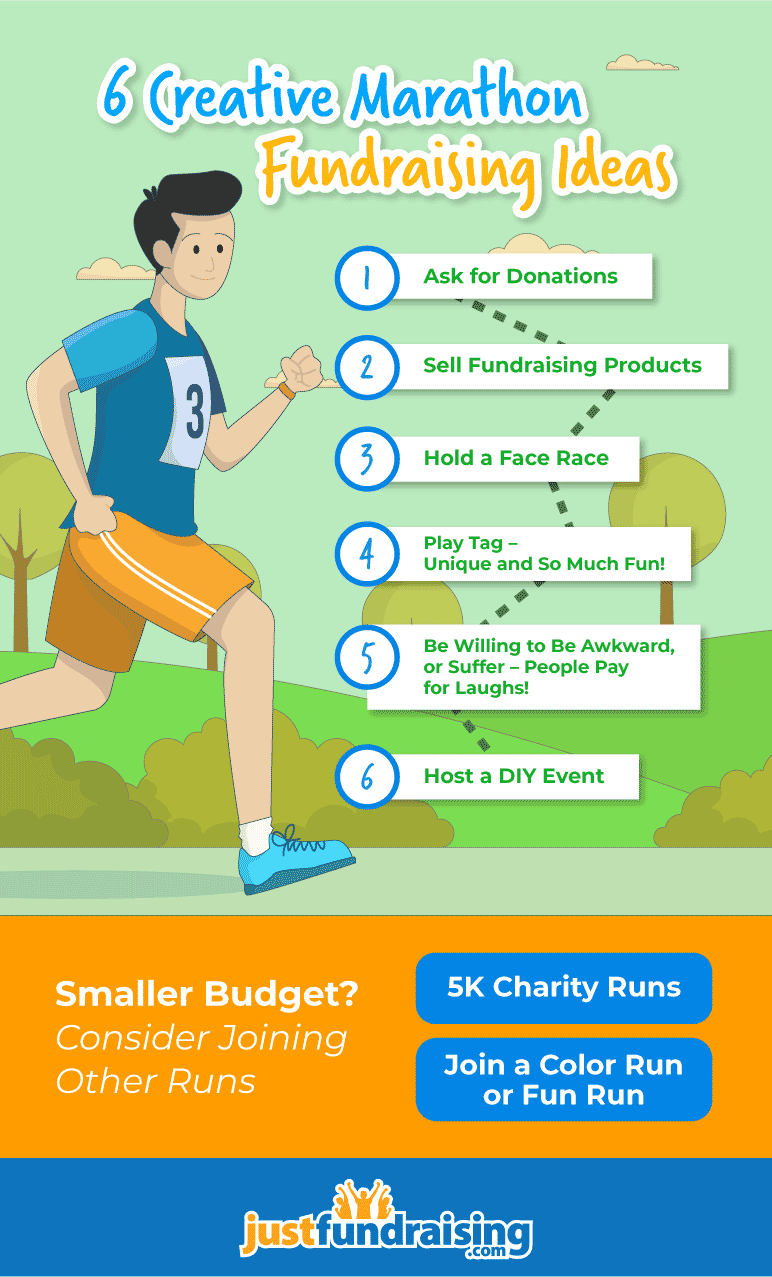The image depicts a vibrant, eye-catching fundraising flyer designed to promote marathon fundraising ideas. Dominating the poster is a cartoon character of a runner, who is animated and whimsical in style. The runner, wearing a green shirt, orange shorts with a white stripe on the side, blue shoes, white socks, a yellow wristband, and a bib numbered three, is seen smiling as he runs on a road flanked by trees, grass, and shrubs.

The headline of the flyer, "Six Creative Marathon Fundraising Ideas," is prominently displayed, with "Six Creative Marathon" in blue and "Fundraising Ideas" in orange. Below the headline, the six suggested ideas are listed in blue numbers, accompanied by green text:
1. Ask for donations
2. Sell fundraising products
3. Hold a face race
4. Play tag, unique and so much fun
5. Be willing to be awkward or suffer, people pay for laughs
6. Host a DIY event

Towards the bottom of the flyer, there is a section encouraging participation in other runs for those with smaller budgets, suggesting options such as 5K charity runs, color runs, or fun runs. The flyer concludes with the website "justfundraising.com" displayed at the bottom, inviting viewers to learn more.